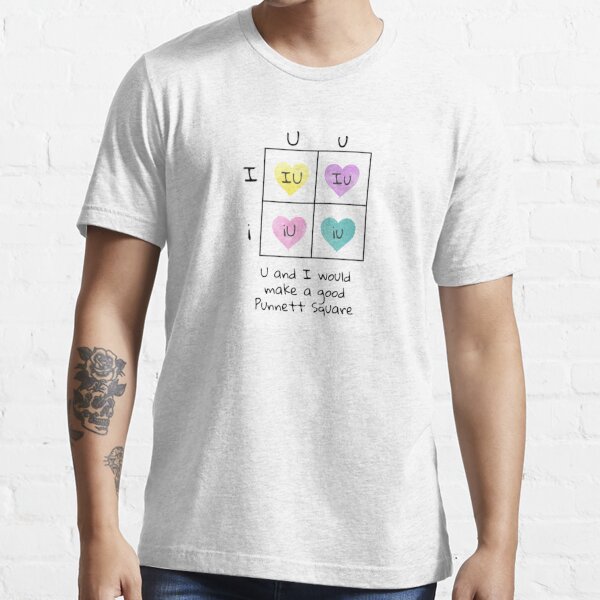The photograph features a man modeling a white crew neck T-shirt with short sleeves. The frame captures him from the bottom of his chin to mid-hip, showing part of his neck and his right forearm. The T-shirt is adorned with a graphic on the chest, structured as a four-square grid. The Y-axis on the left features a capital 'I' at the top and a lowercase 'i' at the bottom. The X-axis along the top displays a capital 'U' in the first column and a lowercase 'u' in the second column. Within each square of the grid, there are hearts with the letters 'IU' in varying color combinations: a yellow heart with 'IU' in the top left, a lavender heart with 'Iu' in the top right, a pink heart with 'iU' in the bottom left, and an aqua-colored heart with 'iu' in the bottom right. Below the grid, black text reads, "U and I would make a good punnett square," humorously playing on the genetic concept. The model's right forearm showcases a detailed black tattoo of a flower that some may find resembles Yoda from Star Wars. He is also wearing dark blue jeans and stands against a light gray background, adding to the minimalist aesthetic of the image.